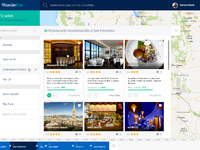This is a screenshot displaying a travel service interface, likely akin to Booking.com, though the small size and poor resolution make it difficult to confirm. The overall layout and elements are discernible despite the clarity issues.

In the central part of the image, there are six smaller images arranged in two rows. These images seem to showcase various landmarks or interiors, though their low resolution obscures precise details:
1. The first image, possibly depicting a fireplace.
2. The second image appears to be a dining room in a restaurant.
3. The third image might show a plate of food.
4. The fourth image could depict a tower that isn't the Eiffel Tower, possibly something like the Space Needle.
5. The fifth image resembles a storefront.
6. The sixth image gives the impression of a nighttime scene, perhaps reminiscent of a medieval fair.

Behind these images, there’s a blurred map, similar to ones found on Google Maps or Apple Maps, suggesting that this interface has geolocation or mapping features.

At the top and bottom of the screenshot are blue bars, which might include navigational elements or areas where users can log into their accounts. The left-hand side of the interface contains various input options like selecting an arrival date, departure date, destination city, and price range, mimicking typical features found in travel booking services.

Overall, while the screenshot provides a basic understanding of the interface’s layout and purpose, the poor resolution significantly limits the observation of finer details.